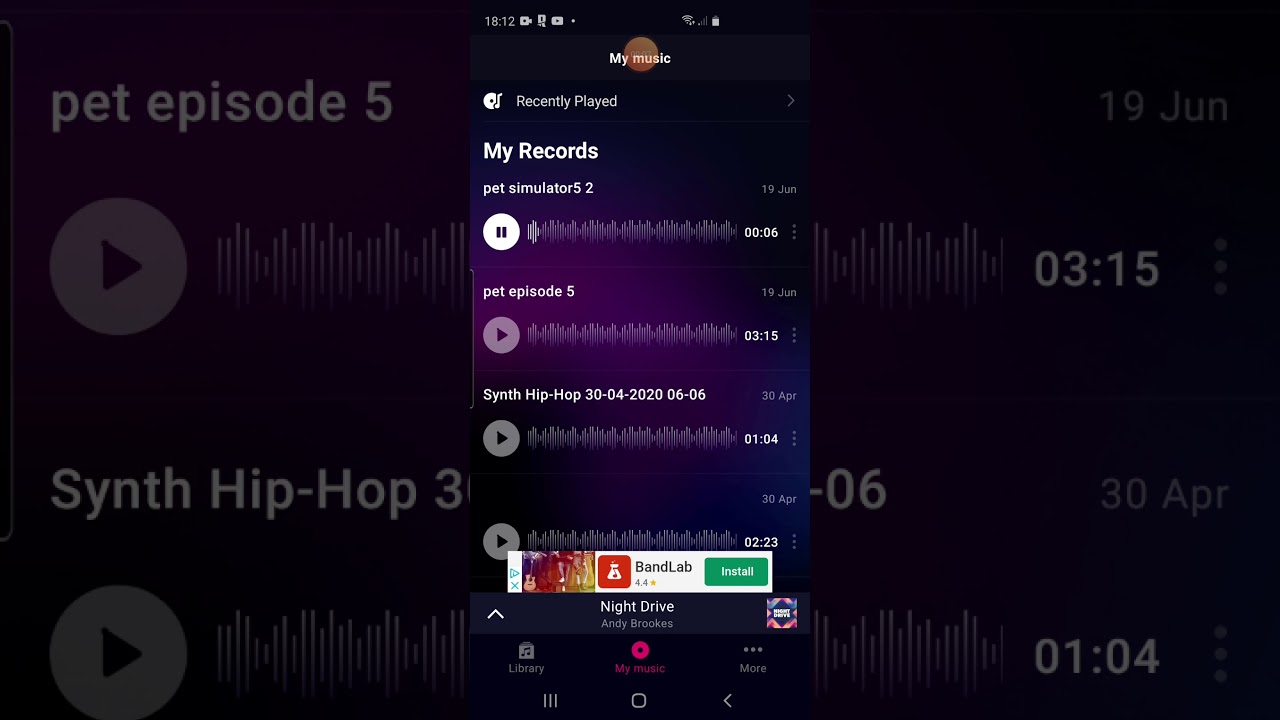This screenshot showcases a music app interface predominantly in dark gray tones with white text and icons. At the top, there's a dark gray bar with a title, "My Music," displayed in white text centered within an orange circle. Directly beneath this title, there is a "Recently Played" button. Below this button lies the "My Records" section, which lists playlist items.

The first item under "My Records" is "Pet Simulator 5.2," featuring an audio player interface equipped with a white pause button. Moving further down, "Pet Episode 5" is listed, accompanied by a play button, time display, and a menu button with three vertical dots on the right side.

Continuing down, the "Synth Hip Hop" entry is dated "30-04-2020, 06-06," and also includes an audio player under it, and another similar player below that. At the bottom of the interface is a Google Ad for "BandLab," featuring a green "Install" button on the right side. 

This concludes the visual description of the music app’s screenshot.